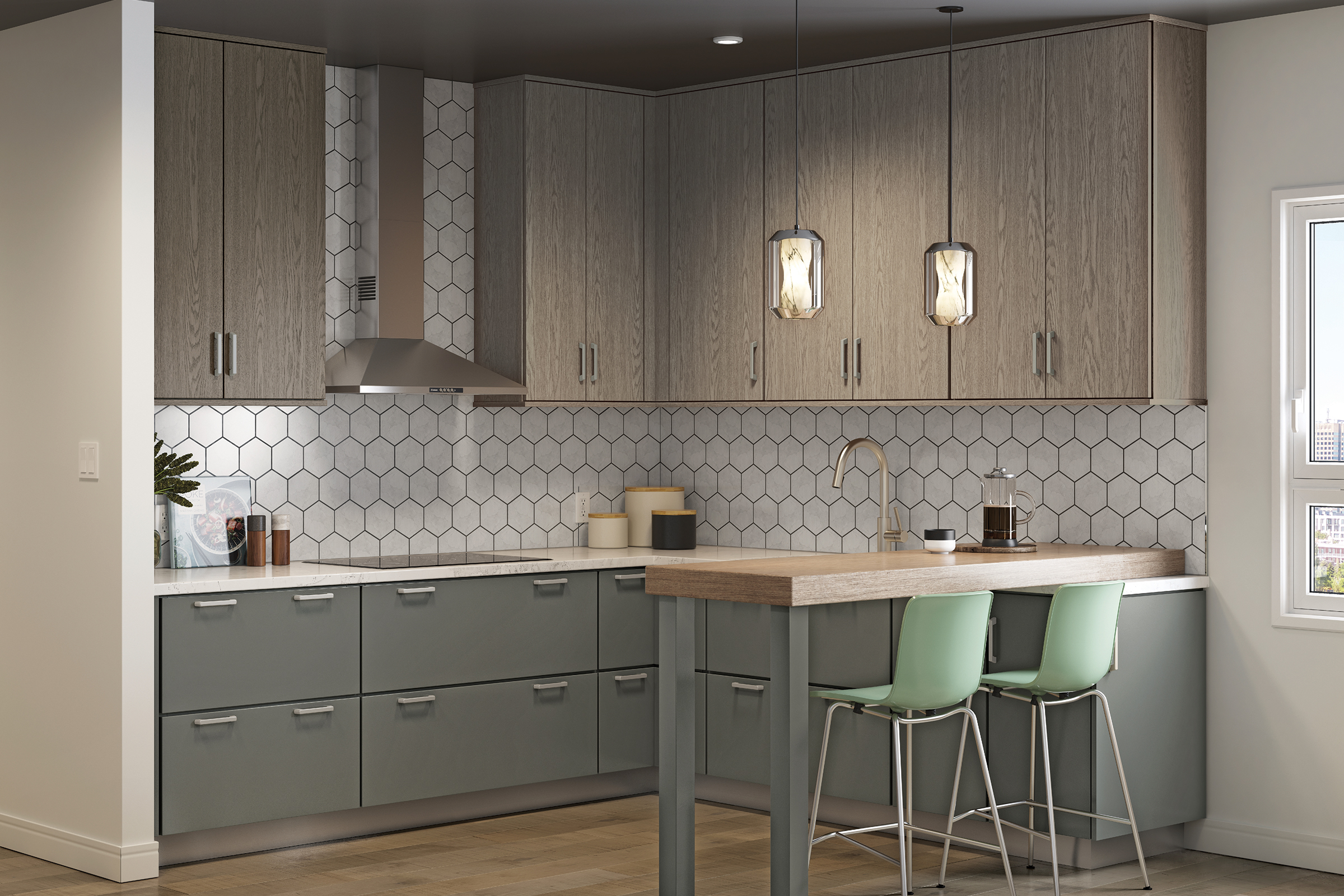This is a detailed image of a computerized kitchen viewed at an angle, featuring an L-shaped countertop made of light-colored stone. The lower cabinets are a gray color, each equipped with two pull-out handles. The backsplash consists of light-colored hexagon tiles with dark grout. A glass-top stove sits beneath a silver vent hood. The upper cabinets are tall with a gray wood grain finish. The kitchen sink, with a brass or champagne bronze faucet, is complemented by a small wooden peninsula extending from the L-shaped counter. This peninsula has two sage green bar stools with silver legs.

On the countertop by the sink, there's a coffee pitcher, which appears to be half-full, and a jar of unknown contents. In the corner, you can find a cookie jar, a sugar jar, and a rice jar. The kitchen features several drawers that resemble office drawers. Hanging lights illuminate the space, though one is lit while the other is not. The ceiling above is dark gray, and a white wall on the left side contains visible switches. On the right, a white-framed window allows natural light to enter, providing a glimpse of some buildings and greenery outside. There are also salt and pepper shakers placed on the countertop.